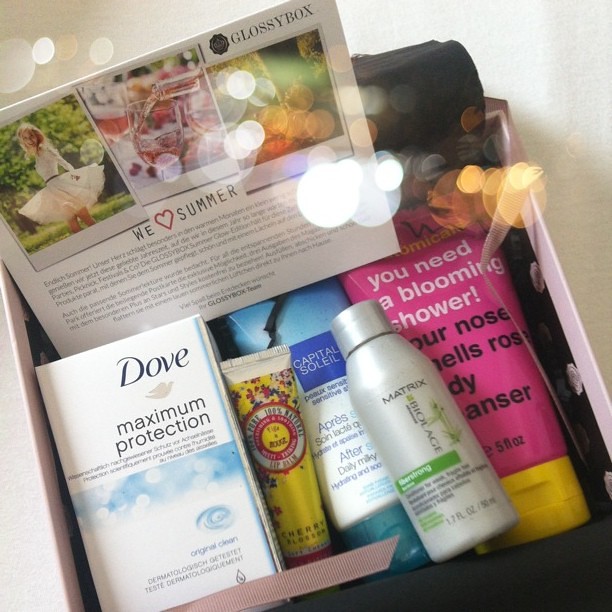The image depicts the interior of a glossy subscription box designed to resemble something from a high-end magazine. Inside, a card is propped up featuring three Polaroid-like pictures, with the words "We ❤️ Summer" and several lines of black text beneath them. The contents of the box are neatly arranged from left to right as follows: a Dove Maximum Protection deodorant, a yellow tube identified as Cherry Blossom Lip Balm, a white and green Capital Soleil bottle, a small travel-sized Matrix Balayage product, and to the far right, a pink bottle with yellow cap and the words "You Need A Blooming Shower" in black and yellow lettering.